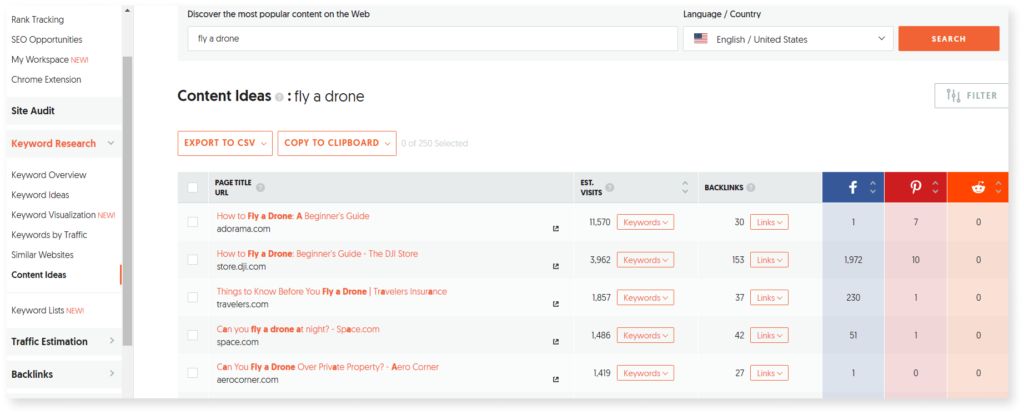Screenshot capturing a comprehensive overview of an SEO and content research platform interface. 

### Left Sidebar
A neatly organized navigation panel is present on the left side, featuring various functional areas:
- **Rank**
- **Tracking**
- **SEO Opportunities**
- **My Workspace** (highlighted with an orange "New" tag)
- **Chrome Extension**
- **Site Audit**
- **Keyword Research** (subheader)
  - **Keyword Overview**
  - **Keyword Ideas**
  - **Keyword Visualization** (highlighted with an orange "New" tag)
  - **Keywords by Traffic**
  - **Similar Websites**
  - **Content Ideas**
  - **Keyword Lists** (highlighted with an orange "New" tag)
  - **Traffic Estimation**
  - **Backlinks**

### Main Body
At the top of the main section, a prominent gray rectangle contains a header and a search bar:
- **"Discover the Most Popular Content on the Web"** serves as the header.
- A search box with the query "Fly a Drone" entered.
- Language and region set to **English, United States**.
- An orange **"Search"** button accompanies the search box.

Below the search bar, a subheading labeled **"Content Ideas: Fly a Drone"** introduces the content insights section. This section includes:
- Two action buttons: **"Export to CSV"** and **"Copy to Clipboard"**, both framed in orange-outlined rectangles.

A gray bar spans horizontally across the page, marking the start of a data table with the headers: **Page Title and URL**, **Est. Visits**, **Backlinks**, and social media columns for **Facebook (blue)**, **Pinterest (red)**, and **Reddit (orange)**.

### Data Table Entries
1. **"How to Fly a Drone: A Beginner's Guide"**
   - Est. Visits: **11,578**
   - Backlinks: **30**
   - Facebook: **1**
   - Pinterest: **7**
   - Reddit: **0**

2. **"How to Fly a Drone: Beginner's Guide"**
   - Est. Visits: **1,962**
   - Backlinks: **153**
   - Facebook: **1,972**
   - Pinterest: **10**
   - Reddit: **0**

3. **"Things to Know Before You Fly a Drone"**
   - Est. Visits: **1,857**
   - Backlinks: **37**
   - Facebook: **230**
   - Pinterest: **1**
   - Reddit: **0**

4. **"Can You Fly a Drone at Night"** by Space.com
   - Est. Visits: **1,486**
   - Backlinks: **42**
   - Facebook: **51**
   - Pinterest: **1**
   - Reddit: **0**

5. **"Can You Fly a Drone Over Private Property"** by Arrow Corner
   - Est. Visits: **1,419**
   - Backlinks: **27**
   - Facebook: **1**
   - Pinterest: **0**
   - Reddit: **0**

This detailed screenshot reveals how the platform facilitates comprehensive SEO and content strategy by offering various tools to analyze keywords, evaluate content performance, and keep track of backlinks and social media metrics.